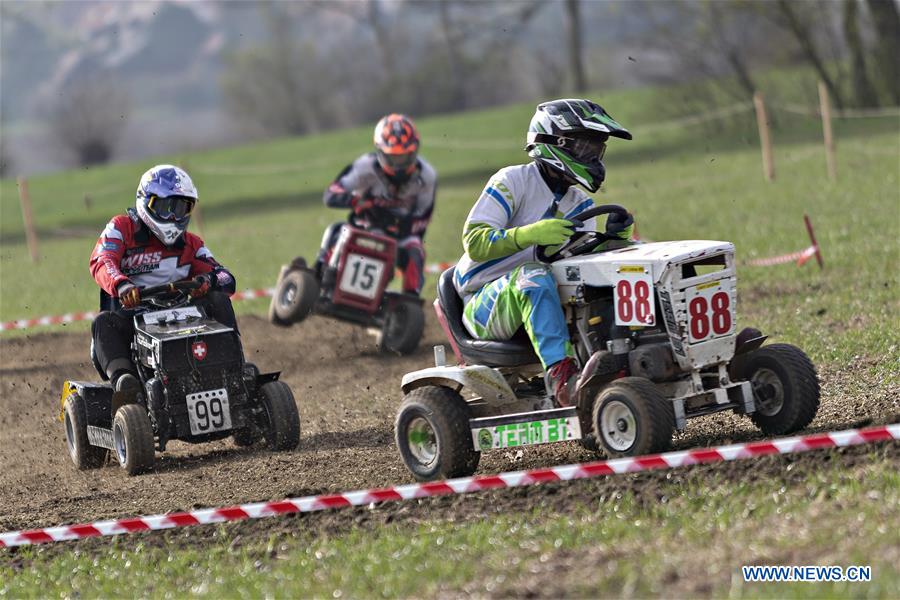The image captures a dynamic daytime race scene involving what appear to be modified lawnmowers, equipped for racing and navigating a track barriered by red and white lines. The setting is an open green field, with patches of brown soil and a backdrop of lush trees and a hill under a sunny sky. There are three racers, each on a distinctively numbered and colorful mini-tractor. Leading the race, the number 88 vehicle is white, driven by a person in a green, white, and blue racing suit with a matching helmet and gloves. Trailing closely behind, the number 99 vehicle is black, with the driver clad in a red jacket, black pants, and a white helmet. The third mini-tractor, numbered 15, is maroon and black, and its driver is wearing a grey and black jacket with a red and black helmet. Noteworthy is that the number 15 vehicle appears to be precariously tilted, indicating a potential flip. All riders are fully equipped with racing gear and helmets, emphasizing the competitive and thrilling nature of this unique race.